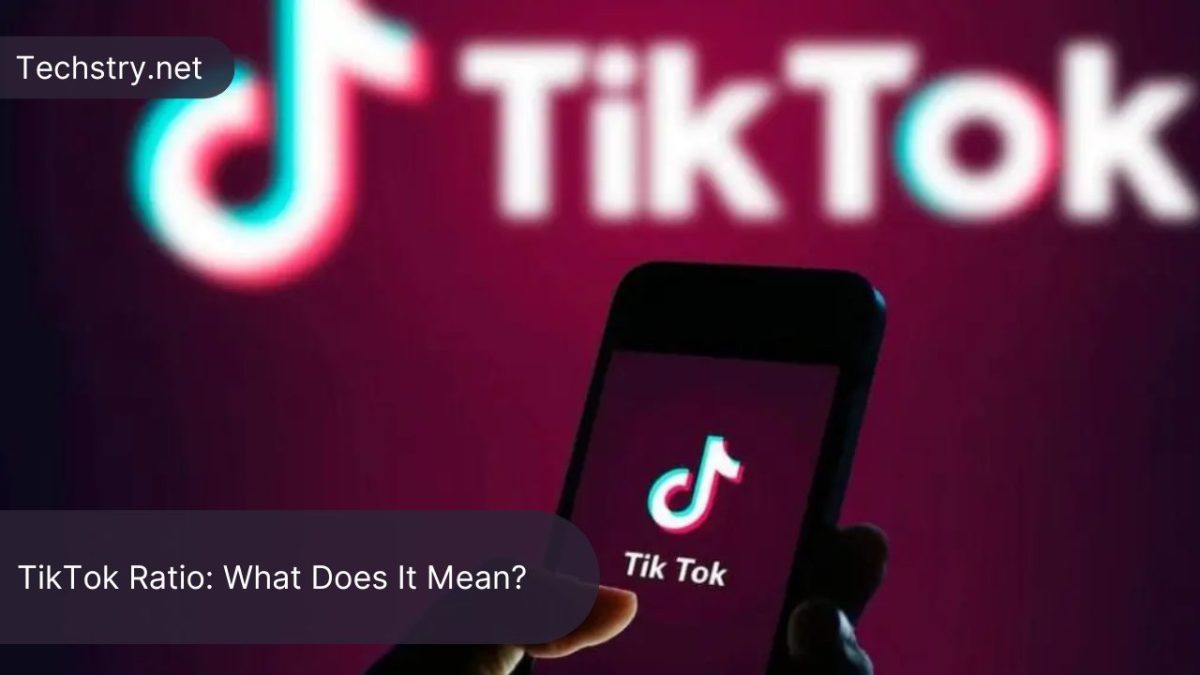This image features a purple square background with prominent design elements. At the top of the square, the TikTok logo and the word "TikTok," both in white, are displayed. Centrally, there is a black oval which contains the text "stream.net" in white. A person is holding a phone in their left hand, and the TikTok app interface is visible on the phone screen. The entire layout conforms to TikTok's standard aspect ratio, ensuring it is optimized for the platform. The overall aesthetic emphasizes TikTok branding and is unified by the monochromatic white elements against the purple and black colors.